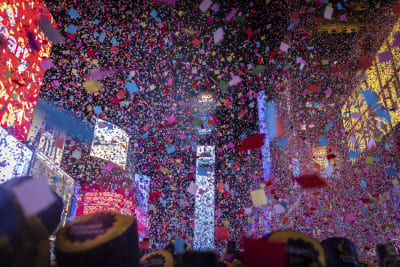This image captures a vibrant New Year’s Eve celebration in Times Square, New York City. The scene is set against a dark night sky, illuminated by an array of brightly lit, animated billboards and signs. A distinctive tall, silver-blue billboard dominates the center, flanked by a red screen on the top left and a yellow sign on the top right. The photograph is angled upwards at about 30 to 45 degrees, capturing the tops of several heads. The people are wearing black, conical hats adorned with yellow squiggly designs and white text, indicative of the coordinated accessories often seen at such events. The air is thick with an overwhelming amount of colorful confetti—red, blue, white, and various other hues—that blurs the details of the signs and adds a festive, chaotic feel to the atmosphere. The colorful square-shaped confetti rains down, creating a sense of excitement and celebration, marking what is unmistakably the moment when the iconic ball drops to ring in the New Year.